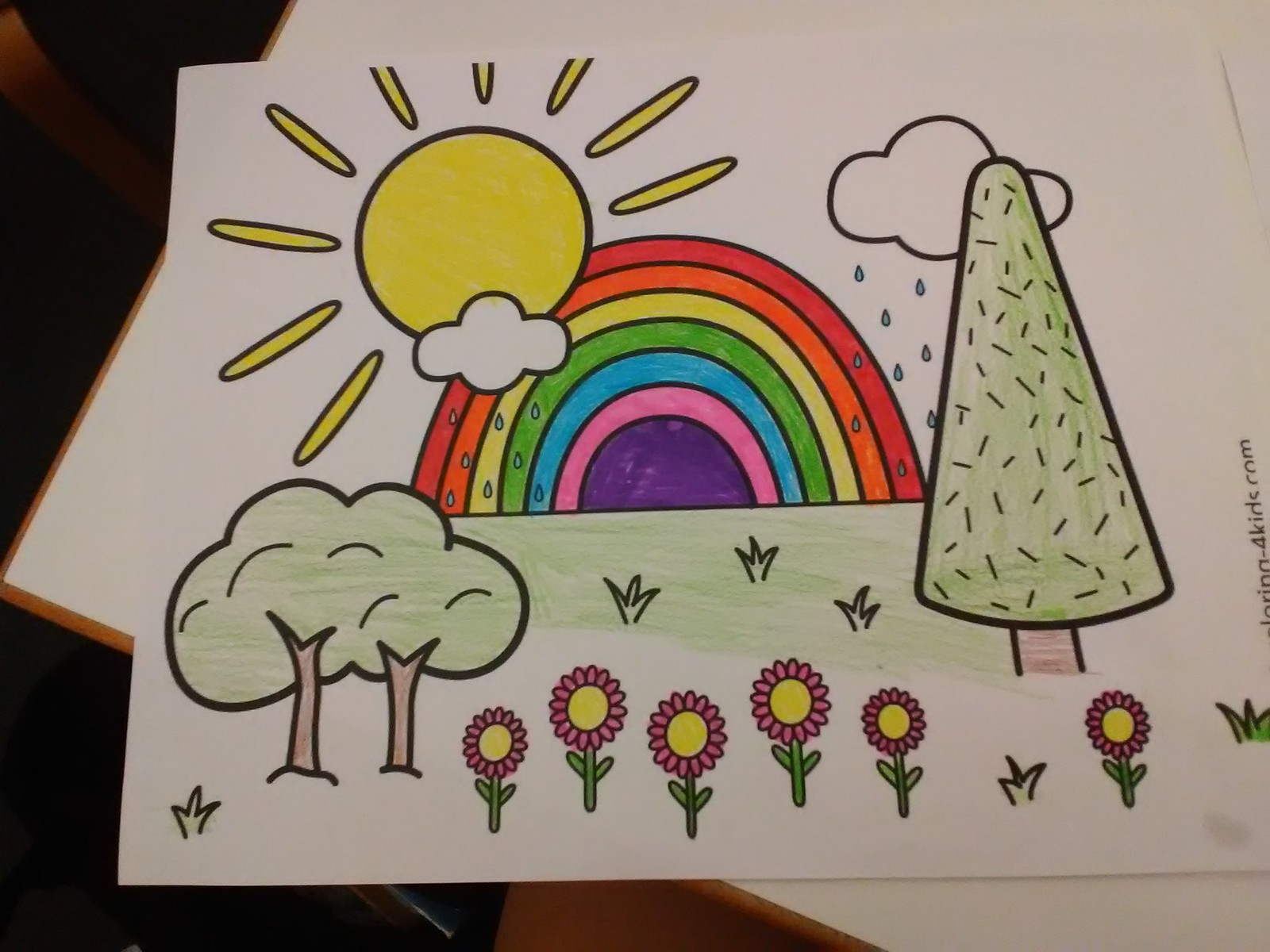This is a detailed image from a coloring book page, primarily colored with crayon. The scene features a vibrant field filled with six flowers, each with green stems, a yellow center, and red petals. The flowers stand on a green lawn, accented with tufts of grass drawn in black crayon, each tuft having three blades of grass. On the left side of the field, there are two trees with brown trunks and mingling green canopies, creating the appearance of a single leafy mass. On the right side, there is an evergreen tree with a short brown trunk and a triangular green top, detailed with little black lines.

In the background, a large rainbow arches over the field, colored vividly with stripes of red, orange, yellow, green, blue, pink, and purple, following the ROYGBIV order. To the top left of the rainbow, a bright yellow sun is partially obscured by a small cloud, from which raindrops are falling. Another larger cloud on the right side, behind the evergreen tree, also releases raindrops. The overall scene is set on an 8 by 10 piece of white paper that lies on a flat, off-white surface, revealing another piece of paper underneath. The entire image is detailed and colorful, capturing a picturesque outdoor setting.